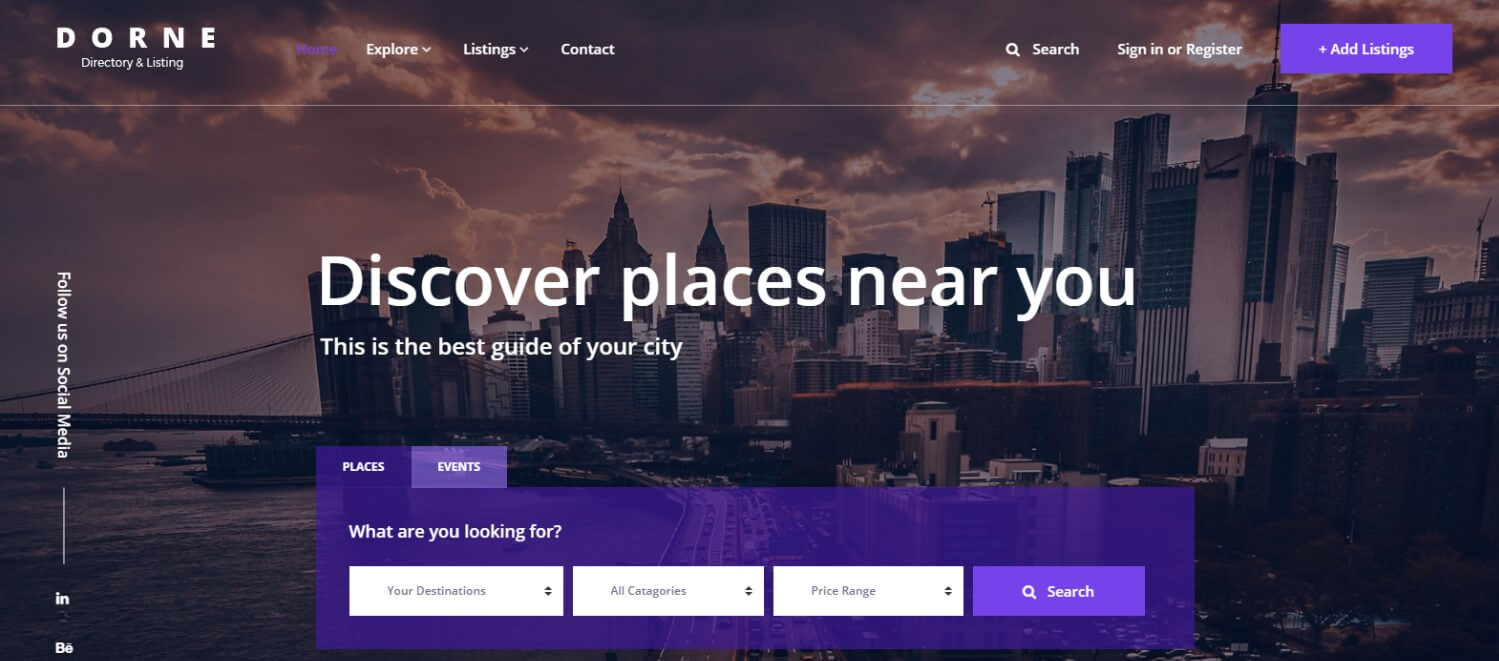The image showcases the homepage of the Dorn Directory and Listing website. The design is minimalist, with a predominantly white background and basic text elements. The navigation bar includes several options in white text: "Explore Listings," "Contact," "Search," "Sign In," "Register," and "Add Listings." The "Home" button appears to be clicked, indicated by a purple hue.

Dominating the center of the page is a bold, white text headline that reads, "Discover Near You," accompanied by the subtext, "This is the best guide of your city." 

On the left side of the page, there is a vertical text aligned under the letter "D" that reads, "Follow us on Social Media," although it's partially truncated and remains incomplete.

The background of the webpage features a stunning photograph of New York City at dusk. The image captures the city's skyline with notable elements like a bridge on the left-hand side, all bathed in a purple dusk hue. The setting sun beams through the clouds, casting a serene glow over the scene. While the focus is on the picturesque elements, the image also includes some less visually appealing parts of the city, adding to its authenticity.